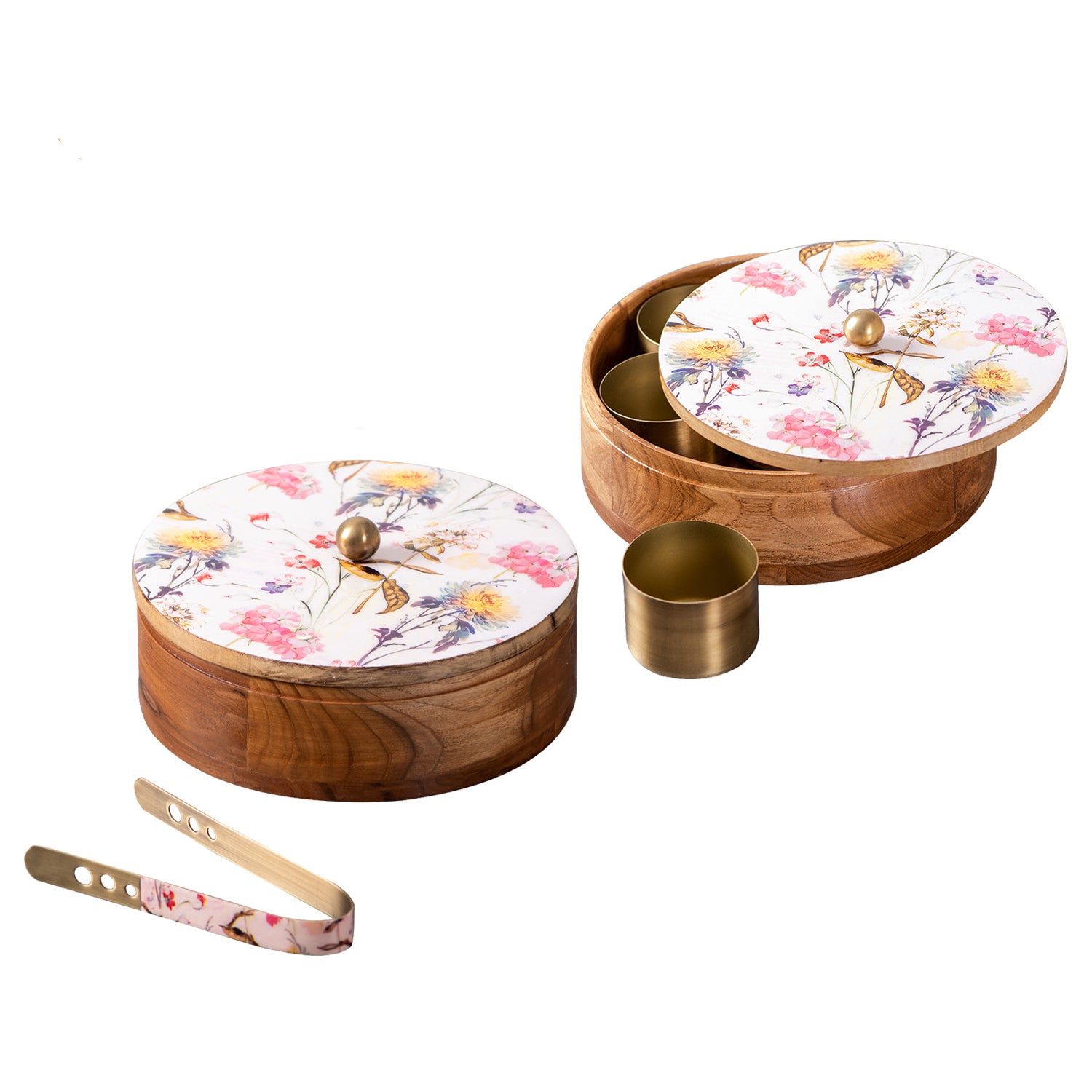The photograph features a set of two charming, circular keepsake boxes crafted from medium-dark wood, each adorned with wooden lids. The lids are topped with decorative bead handles and feature a delicate flower-patterned design against a backdrop reminiscent of floral wallpaper. One box is open, revealing several small, copper-colored cylindrical containers inside, suggesting uses such as holding buttons or tea leaves. The image, likely intended for a product page with its transparent white background, also includes a pair of tongs that share the same floral motif as the lids of the boxes. The copper containers inside the open box do not have lids, and the overall arrangement hints at a capacity for seven or eight such containers in total. The boxes are aesthetically pleasing, blending elements of traditional craftsmanship with practical storage solutions.